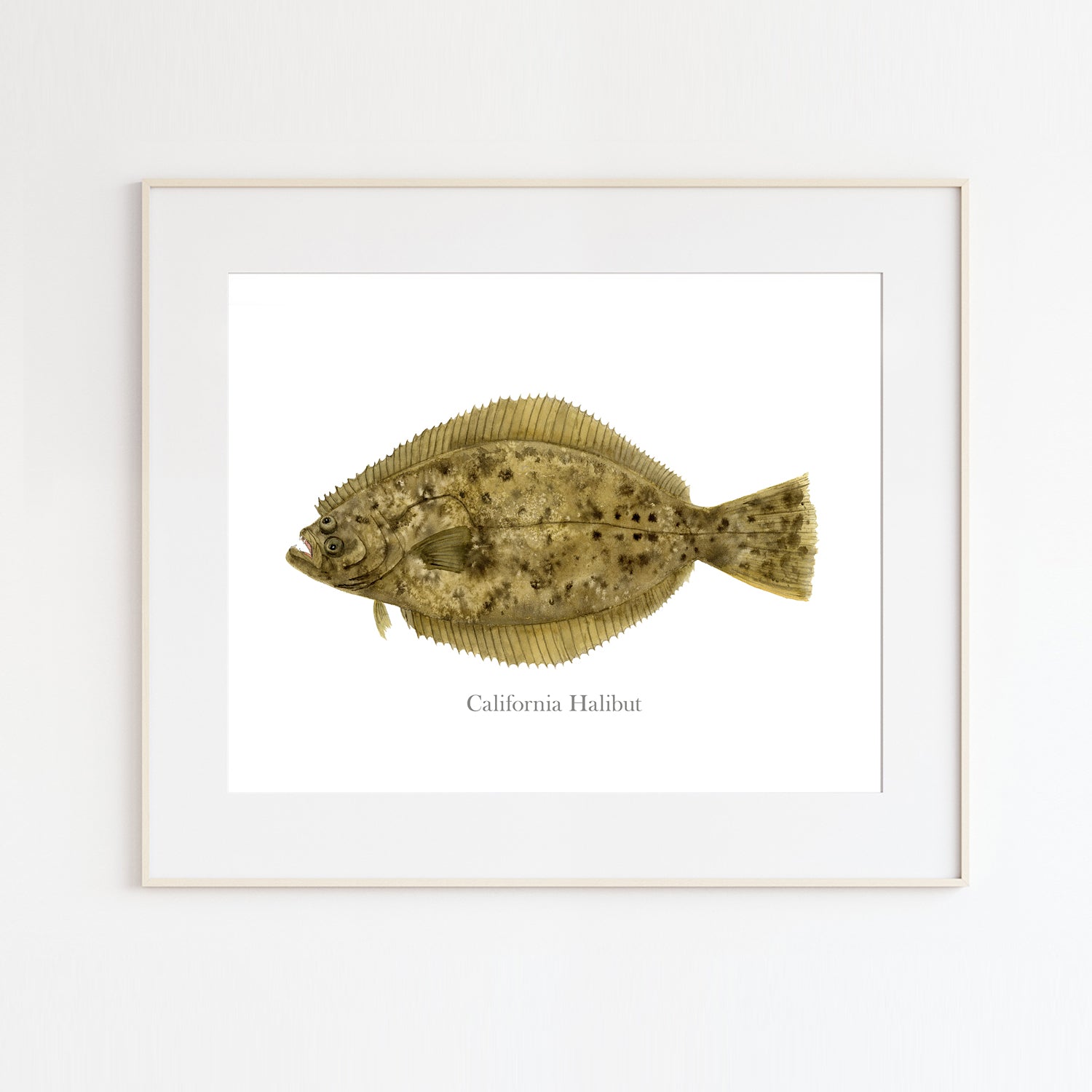The image features a highly detailed, realistic illustration of a California Halibut, centrally positioned on a bright white background. The fish is rendered in brown hues with black spots dotted across its body, capturing the distinctive texture and coloration of the species. The California Halibut's two prominent eyes are situated on one side of its body, indicative of its flatfish nature, and its mouth is slightly open. The fish's fins are jagged and extend from above its eyes down to its tail, which is triangular in shape. Surrounding the image is a light blue matting, framed by a thin, creamy-white or light brown frame. The bottom of the illustration features grey text that reads "California Halibut," providing a clear, concise identification of the subject. The entire framed picture rests against a grey or light blue background, emphasizing the stark contrast and bringing attention to the finely detailed artwork.